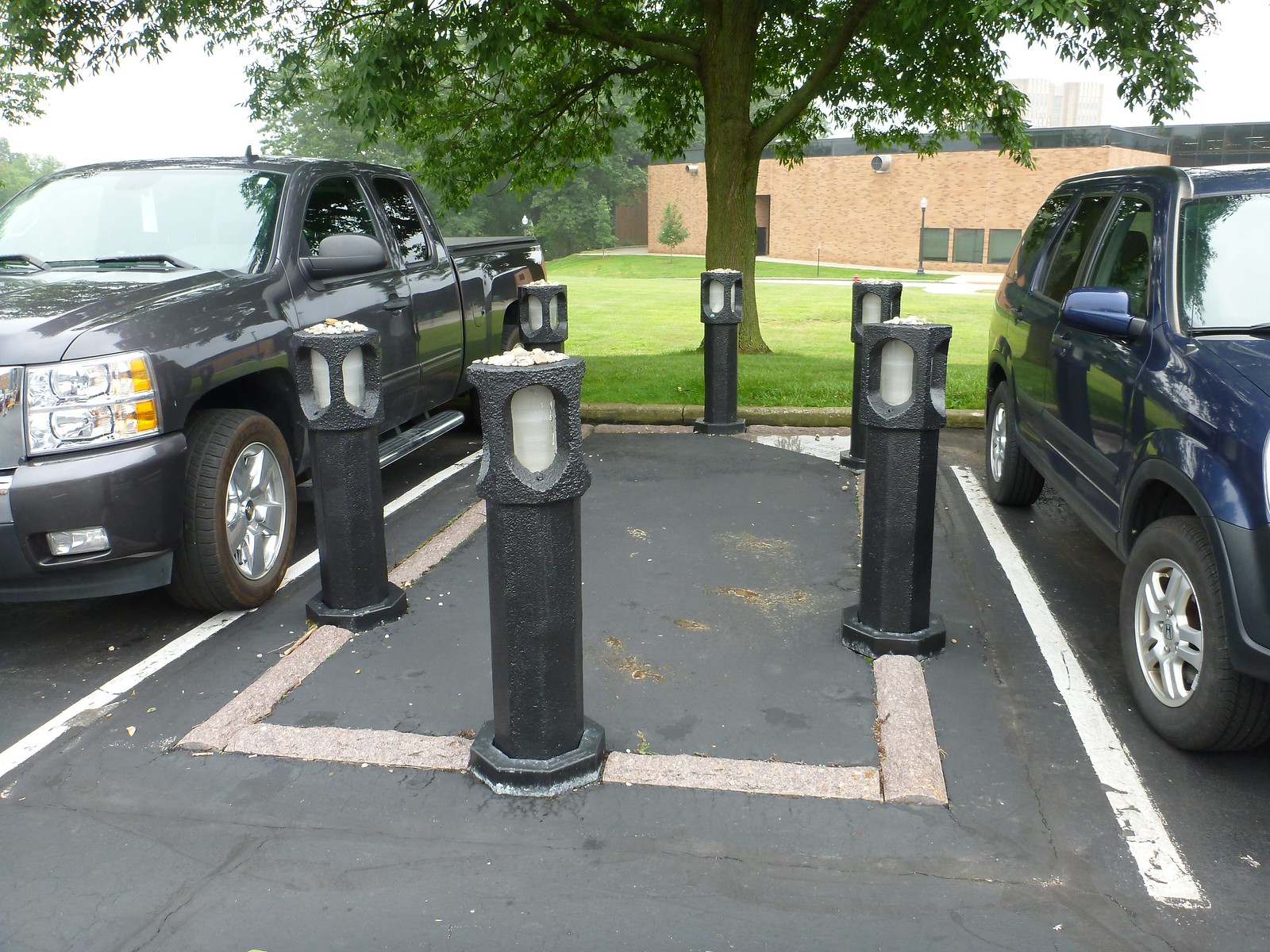This image captures a parking lot featuring two parked vehicles: a black pickup truck on the left and a dark blue SUV on the right. The central parking space between the vehicles is blocked off by six concrete structures resembling lamp posts or bollards. These structures, standing in a circular arrangement, might serve as light sources or reflectors for nighttime illumination. In the background, there is a large tree with lush, dark green leaves and an expansive grassy area that leads up to a one-story brick building, possibly a school. Further back, a few taller residential buildings are visible, albeit through a white, foggy sky, adding a misty ambiance to the scene.